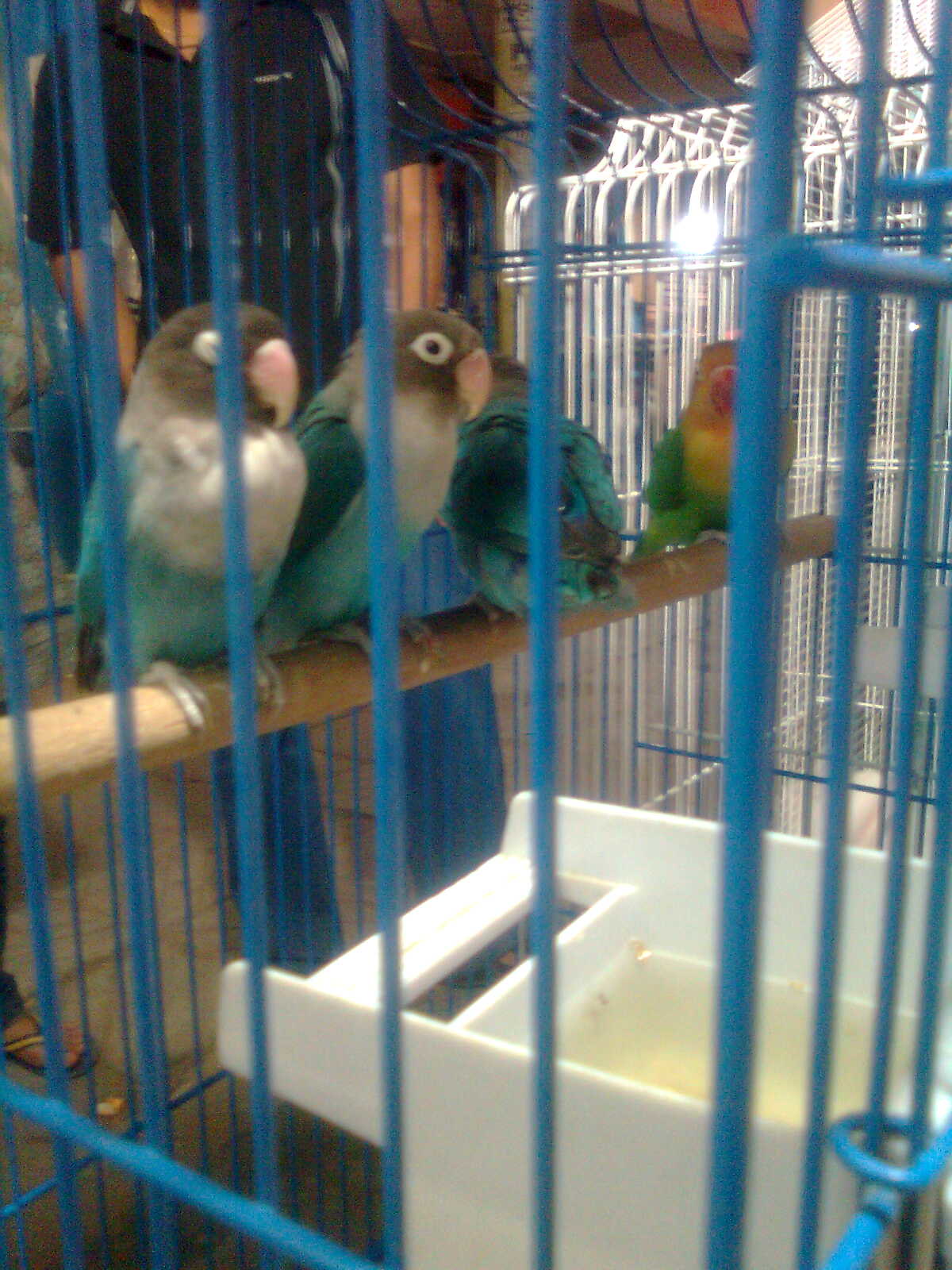The photograph, taken in portrait orientation, depicts a close-up scene of a metal birdcage in vibrant aqua blue. Through the wire bars, which add a textured grid to the image, one can glimpse a person standing behind the cage, though their head is cropped out of the frame. Inside the cage, a light brown, wooden perch extends from the left to the right side, hosting four small, parrot-like birds.

Three of the birds share similar markings: they have a dark brownish-grey head, striking white chests, and vivid turquoise feathers on their backs and wings, with a subtle greenish-blue hue on their lower bodies. The two birds nearest the camera face forward, showcasing their light orange beaks and expressive, white-rimmed eyes with dark pupils. The third parrot faces away, revealing only the turquoise and dark grey tips of its tail feathers. The fourth bird, slightly hidden behind a vertical wire bar, exhibits a unique combination of green lower body feathers and a yellow chest, with hints of yellow, tan, and possibly red on its head.

Below the perch, a white, square-shaped bowl likely containing water is placed on the ground. In the left corner of the image, the photograph captures a person's foot, and their upper body is partially visible towards the top left. Additional white birdcages are faintly seen in the blurred background, suggesting the setting might be a pet shop. The intricate details and vibrant colors of the birds, coupled with the soft blur of the background, draw attention to the serene yet lively scene within the cage.